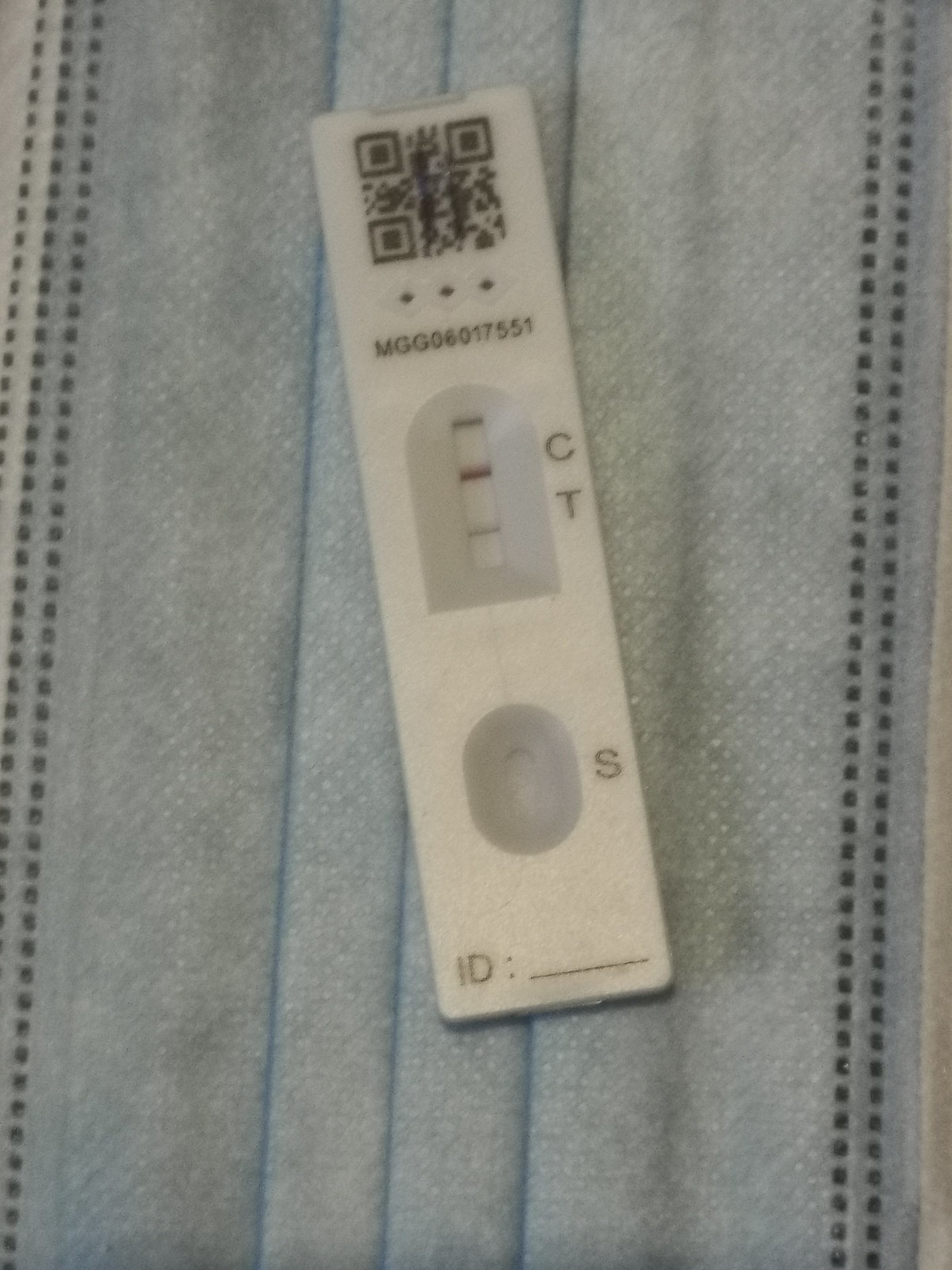The image depicts a slightly grainy photograph of a COVID-19 test kit centered within the frame, which is roughly 30% taller than it is wide. The test kit itself is an off-white, long rectangular piece of plastic with rounded edges, approximately four to five times taller than it is wide, and positioned at an angle as if pointing to 11:30 on a clock. 

At the top of the kit is a black QR code, which likely provides directions or additional information when scanned. Directly below the QR code are three small circular indentations, whose purpose is unclear but could potentially be lights or indicators. Below these circles is a printed alphanumeric code, "MGG 0601751," somewhat discernible despite the image quality.

The body of the test kit features a recessed archway area that is rectangular with a squared-off bottom and a circular top. Within this recessed space are two lines: the line next to the letter "C" is marked with a distinct red color, indicating the control line, while the line next to the letter "T" is faint gray, indicating the test line.

Below the archway is a horizontal oval indentation with a smaller recessed area inside it, labeled with the letter "S" to its right. This area is currently empty.

In summary, the detailed visual depiction describes the various components of the COVID-19 test kit and provides insight into its layout and markings.